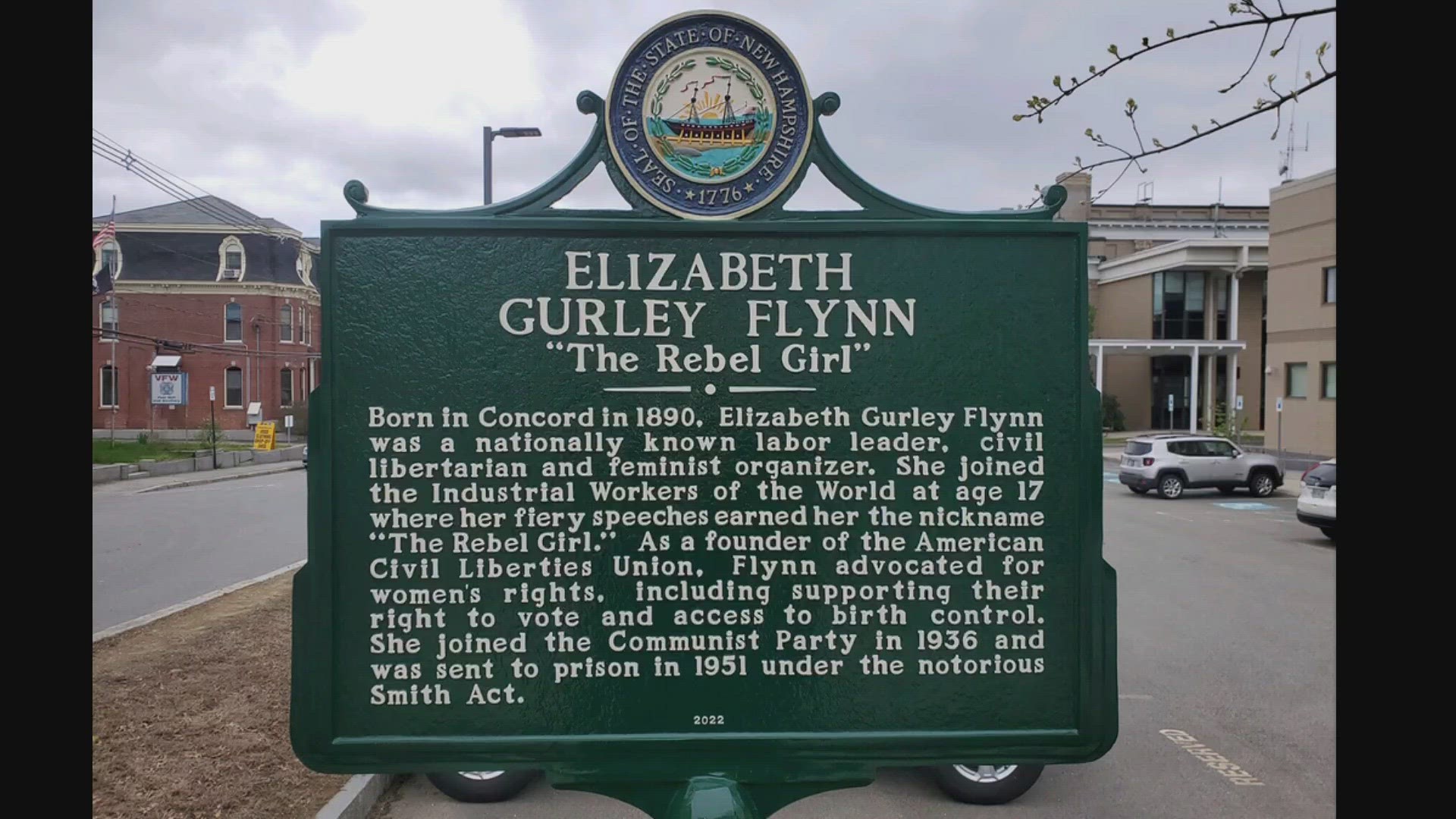This photograph captures a historical site sign located in a small town backdrop featuring a notable brick courthouse and various older buildings, likely from the 1950s. In the median near the road, the green wooden sign prominently displays the Seal of the State of New Hampshire, dated 1776, which features an image of a ship. The sign commemorates Elizabeth Gurley Flynn, known as "the Rebel Girl." Born in Concord in 1890, she was a nationally recognized labor leader, civil libertarian, and feminist organizer. At the age of 17, Flynn joined the Industrial Workers of the World, where her passionate speeches earned her the nickname "the Rebel Girl." She was also a founding member of the American Civil Liberties Union and a staunch advocate for women's rights, championing the right to vote and access to birth control. In 1936, Flynn joined the Communist Party, which led to her imprisonment in 1951 under the Notorious Smith Act. The scene also includes elements such as cars and additional buildings in the distance, underscoring the historical and small-town atmosphere of the location.